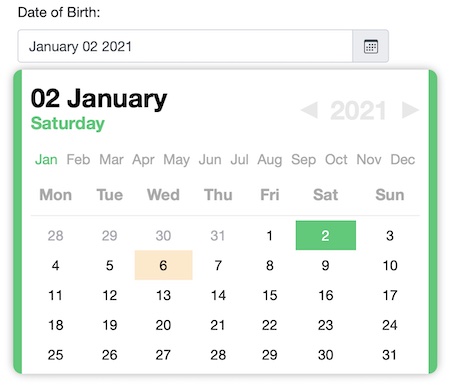### Detailed Caption for Image

The image features a date-related interface on a white background, prominently showcasing a segment that focuses on the date of birth. 

At the top of the image, the phrase "Date of Birth" is displayed in black text with the initial letters "D" and "B" capitalized. Following this text are three ellipses (...), leading into a blank space. 

Below this section, there is a rectangular outline in gray. The right-hand part of this rectangle is shaded in a darker gray. Within this outline, the specific date "January 02, 2021" is written in bold black text. 

Additionally, there is a calendar within the gray rectangle. The calendar itself has a white background with green strips running vertically along its left and right sides. 

In the top left-hand corner of the calendar, "02 January" is written in bold black text with the "J" in January capitalized. Directly beneath this, the word "Saturday" appears in green with a capital "S." On the right-hand side of this section, "2021" is printed in gray flanked by two triangles; one pointing left and the other pointing right.

The next row starts with the abbreviation "Jan" for January in green on the left side, while the rest of the months are abbreviated and displayed in gray: "Feb" for February, "Mar" for March, "Apr" for April, "May" for May, "Jun" for June, "Jul" for July, "Aug" for August, "Sep" for September, "Oct" for October, "Nov" for November, and "Dec" for December.

Below the months, there is some white space followed by the days of the week listed in bold gray text. The abbreviations for the days are as follows: "Mon" for Monday, "Tue" for Tuesday, "Wed" for Wednesday, "Thu" for Thursday, "Fri" for Friday, "Sat" for Saturday, and "Sun" for Sunday.